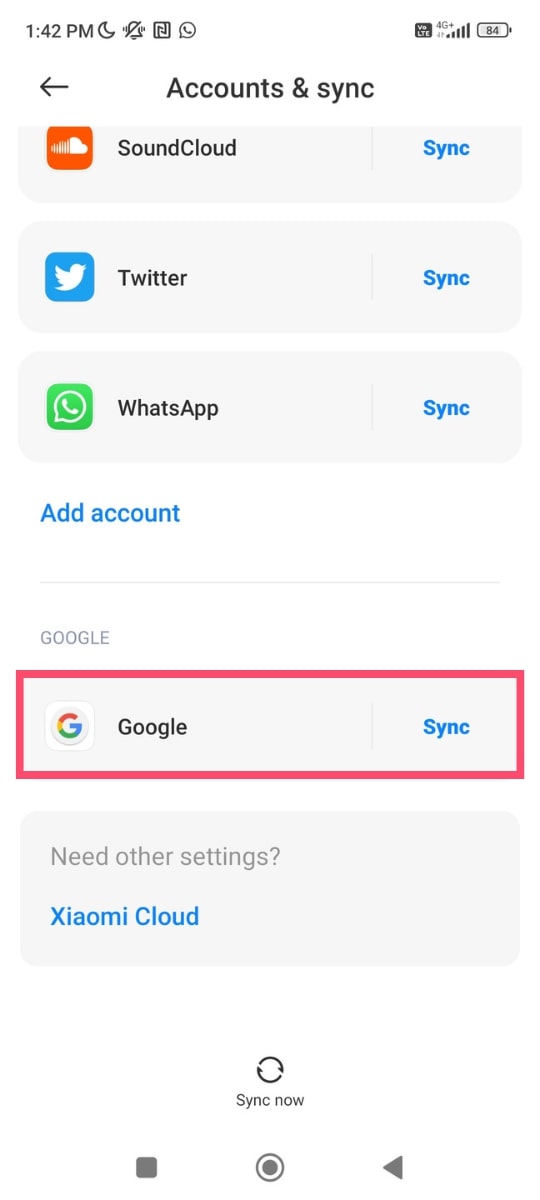This image is a detailed screenshot from a cell phone. In the top left corner of the screen, the time reads 1:42 p.m. There are several status icons to the right of the time: first, a half-moon icon, followed by a circle with a diagonal line through it, an "N" inside a box, and a bubble containing a phone icon. On the far right side, a gray box displays a signal strength icon with five bars and a battery icon oriented sideways, whose battery level is indeterminate due to small text size.

Below these status icons, there's a left-facing arrow on the far left. In the middle of this section, "Accounts in sync" is displayed in gray text. Beneath this, a list of apps and their sync statuses is shown:

- "SoundCloud" in gray, with "Sync" in blue to the right.
- "Twitter" in gray, with "Sync" in blue to the right.
- "WhatsApp" in gray, with "Sync" in blue to the right.

Below these entries, "Add account" is written in blue text. Further down, "Google" is labeled in gray, accompanied by Google's colorful "G" logo, and next to it is a blue "Sync" text inside a red-outlined box.

At the bottom, there's an option labeled "Need other settings" in gray, followed by "XIAOMI Cloud" in blue text.